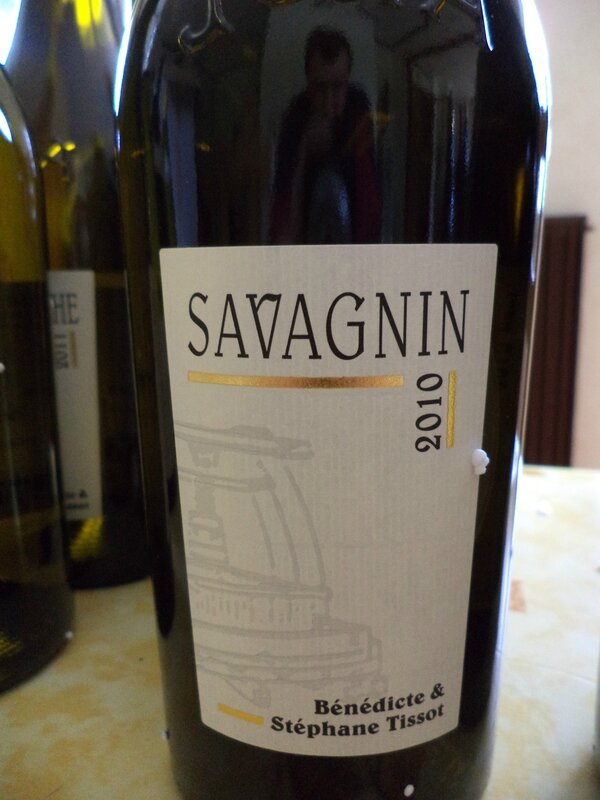In the image, we see a close-up of a dark green Savion wine bottle, positioned on a white table. The white label on the front prominently features "Savion" written in black uppercase letters at the top. Below this, a shiny gold foil horizontally spans across the label, with "2010" inscribed next to it. Beneath the gold foil, there is a faint light gray illustration that seems to depict a wine barrel or some related apparatus. The label further includes the names "Benedict and Stéphane Tissot," written in black text, with another horizontal gold stripe adjacent to "Stéphane Tissot." Flanking the central bottle, two other bottles of wine with similar labeling are partially visible, suggesting they belong to the same product line. The image is so zoomed in that the top of the bottle is cut off where it starts to round into the neck, and the base is almost visible but not completely shown.